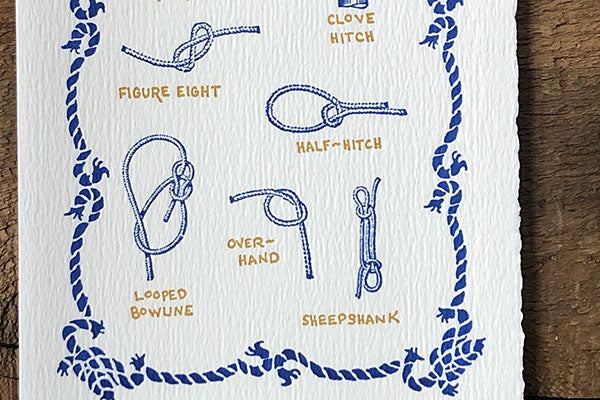This image features a textured, rough piece of white paper set against a dark, untreated wooden background. Illustrated on the paper are six different types of knots, each meticulously drawn in blue. These knots include the Figure Eight, Half Hitch, Looped Bowline, Overhand Knot, and Sheepshank, with a partially visible Clove Hitch in the upper right corner. Each knot is labeled in orange text, enhancing their visibility. Surrounding the paper is a decorative border made of blue ropes, creating a repeating pattern that frames the entire image. The outer ropes feature additional knots in the corners, emphasizing the theme of rope tying. The detailed diagrams show how each knot looks when complete, without providing step-by-step instructions. The overall presentation effectively highlights different methods of tying ropes, focusing on the visual aspects and final appearance of each knot.